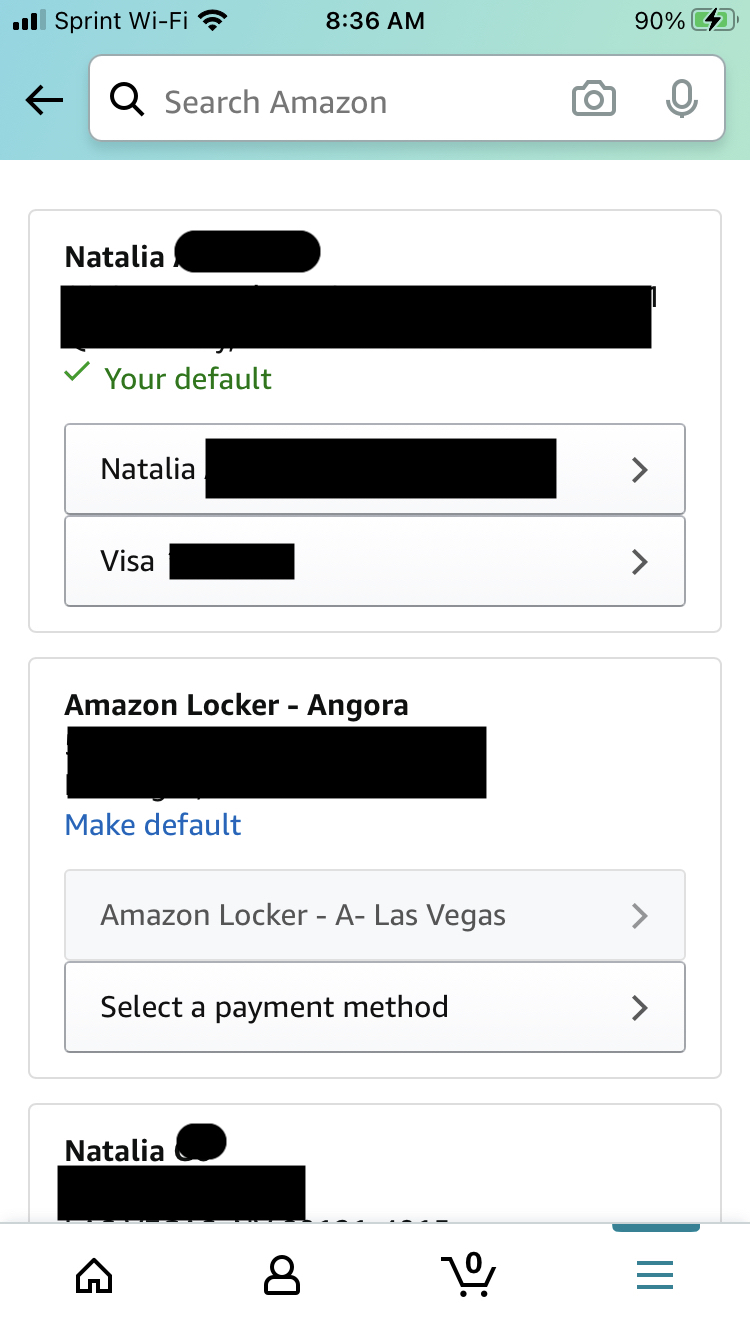The image is a screenshot taken from a cell phone interface. At the very top of the screen, there is a gradient banner transitioning from pale blue on the left to pale green on the right. The left side of the top banner displays "Sprint Wi-Fi" next to icons indicating cell signal and Wi-Fi signal strength. Centrally located is the time, "8:36 AM," and a battery icon showing 90% charge.

Below the banner, there is a left arrow, followed by a search bar with the placeholder text, "Search Amazon." The search bar is accompanied by icons of a magnifying glass, a microphone, and a camera. 

The main content area below the search bar features a white background bordered by a thin light gray line. Displayed prominently is the name "Natalia" with the last name obscured by a crossed-out effect, except for the capital "N." Adjacent to the name is a green checkmark, and the text "your default" appears in gray.

Underneath this section, "Natalia" is repeated, with the last name again obscured. Below, "Visa" and the card number are also crossed out. Further down, there is another bordered section with a square frame, labeled "Amazon Locker-Angora," followed by the obscured information. Beside this, "Make Default" is written in blue text.

The next section lists "Amazon Locker-Las Vegas," followed by the instruction "Select Payment Method." The name "Natalia" appears again with the associated info blocked out.